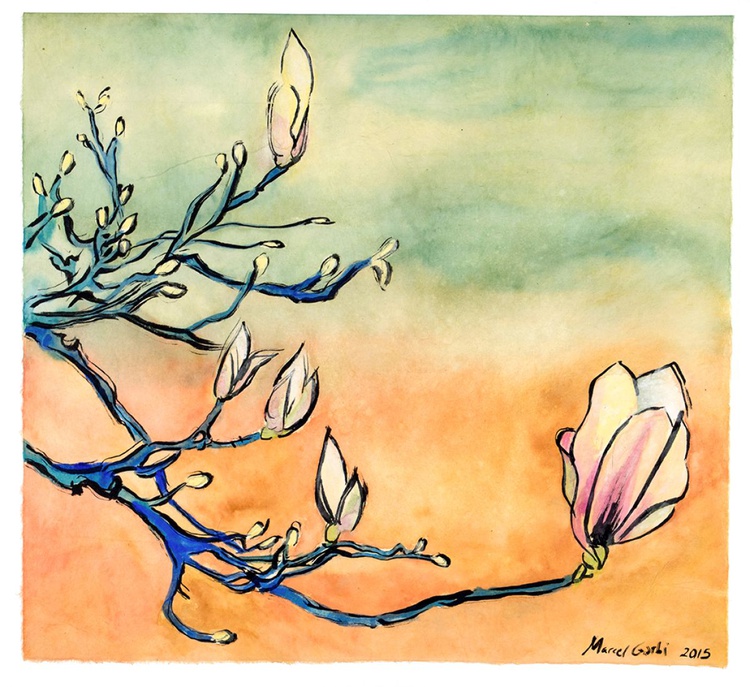The image is a vibrant painting by Meryl Garvey, dated 2015. The background transitions from an abstract blend of green and yellow at the top to brighter orange and yellow hues at the bottom, creating a melded gradient effect in the middle. The focal point is a blue or tealy-green branched plant extending from the left across the painting. A particularly long branch at the bottom features a significant, partially bloomed flower near the right side, with beautifully shaded pink, peach, and yellow petals. Smaller branches, also blue, bear a mix of tiny flowers in shades of pink and peach and numerous yellow buds at their tips. The composition is lush with pastel colors, enhancing the lively and dynamic essence of the artwork.